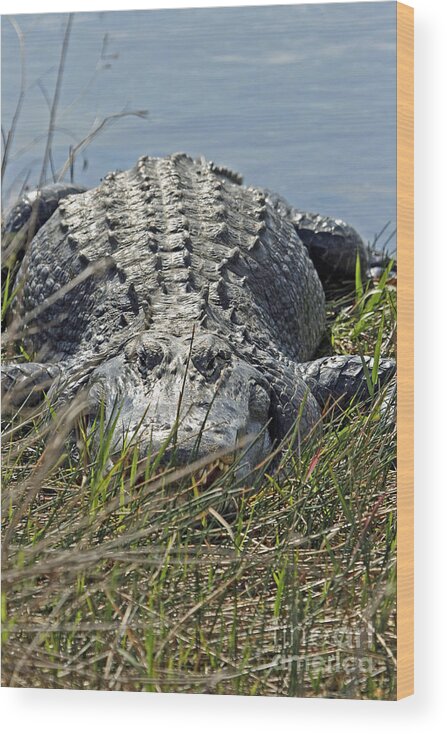This detailed photograph captures a close-up of a large crocodile or alligator lying on a grassy shore with sparkling blue water behind it. The powerful reptile, appearing gray with a shiny back reflecting sunlight, has its eyes half-closed, giving it a relaxed yet watchful demeanor. Its mouth is slightly open, revealing some teeth that are partially obscured by sparse grass and dead twigs. The crocodile’s front arms are splayed out to the sides, and its midsection appears robust and healthy, showcasing prominent ridges along its back. Wooden boards are visible along the edge of the image, adding a rustic frame to this compelling scene of nature.